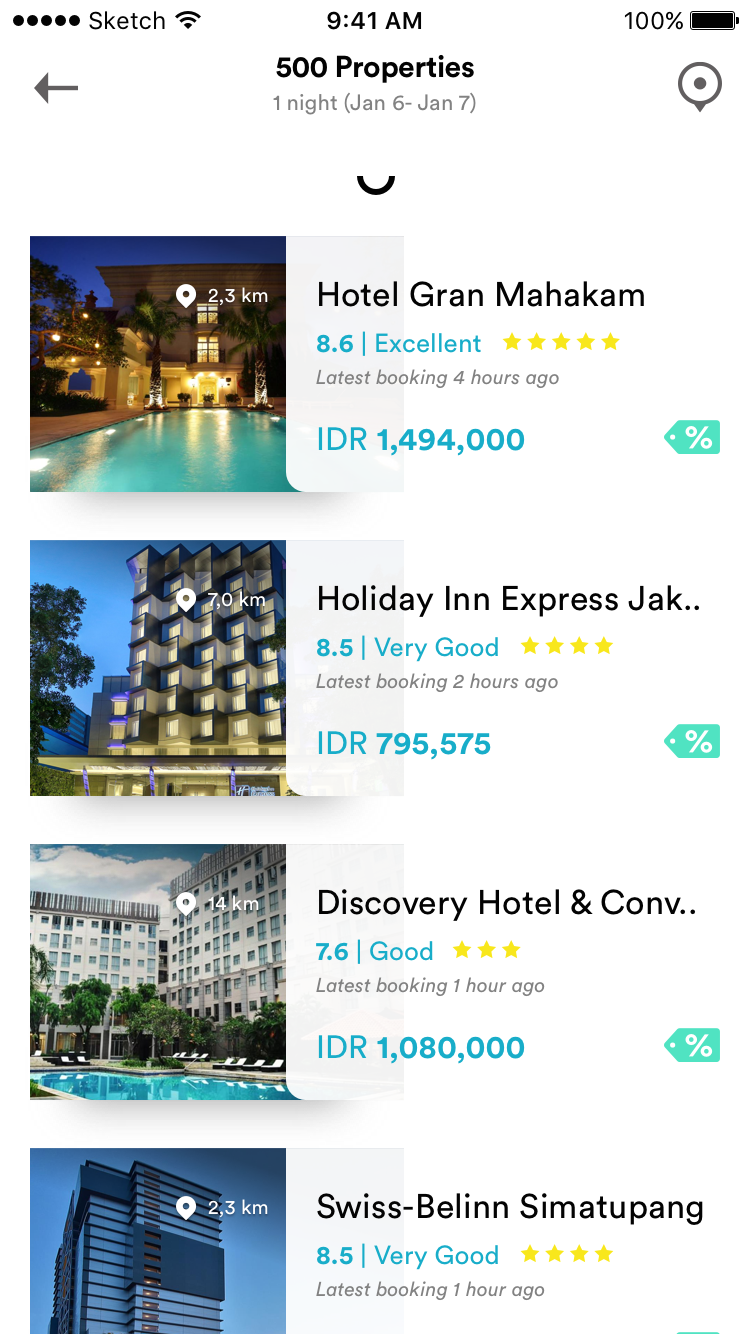This is a detailed description of a smartphone screenshot showcasing properties available for booking:

At the top of the screen, there are five black dots followed by a sketch icon and a Wi-Fi icon. The time displayed in the middle of the status bar is 9:41 AM, and the battery is fully charged at 100%. Below the status bar, there's a navigation section with a left-facing arrow on the left side and a text in the center that reads "500 properties, one night" with the dates "(January 6th - 7th)" in parentheses, and a location icon next to it.

The main section of the screen features various hotel listings starting with images:

1. **Hotel Grand Mahakam**: The first image is of the outdoor pool area of the hotel. It has a high rating of 8.6 stars. The latest booking was made four hours ago. The cost per night (ADR) is IDR 1,494,000.

2. **Hotel Inn Express**: The second image shows the hotel's exterior at dusk, with lights illuminating the room windows. The rating is 8.5 stars, the latest booking happened two hours ago, and the cost per night is IDR 795,575.

3. **Discovery Hotel and Conference Center**: The third image is of another pool and the hotel’s facade. It has a rating of 7.6 stars (category: good), with the latest booking occurring one hour ago. The cost per night is IDR 1,080,000.

4. **Swiss-Belhotel Simatupang**: The fourth image features the hotel building's top floors captured at dusk. This property has an 8.5-star rating (very good) and was last booked an hour ago.

This descriptive caption provides a clear and detailed overview of the smartphone screenshot, specifying the visual elements, ratings, booking details, and prices associated with each hotel listing.